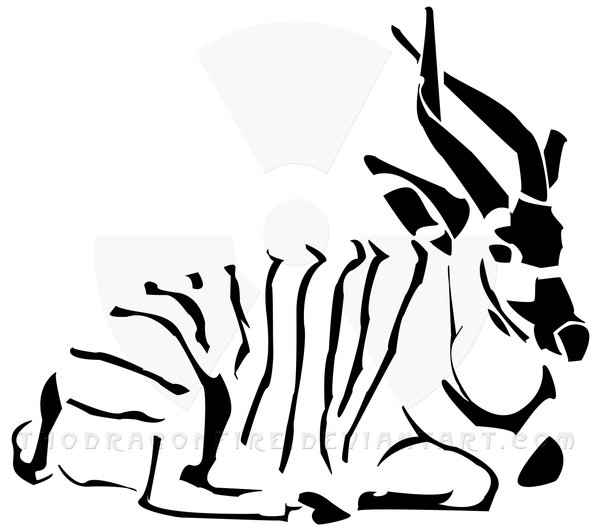The image is a minimalist ink cutout print of an ibex or an antelope-like creature, possibly a new type of African gazelle. The creature's defining features are highlighted in black on a stark white background, showing only the dark areas. It has long, curved horns, black points on its face including its nose and eyes, striped markings along its back, distinct black hooves, and pointed ear tips. The gazelle is depicted in a sternal resting position with its short tail behind it.

Embedded faintly in the middle of the gazelle's body is a radiation hazard symbol, giving the image an unusual twist. Beneath the creature, there's a barely legible watermark, presumably the artist's website, ending with ".com." The watermark is in a faint silver or gray color, blending into the black outlines of the gazelle, making it hard to decipher.